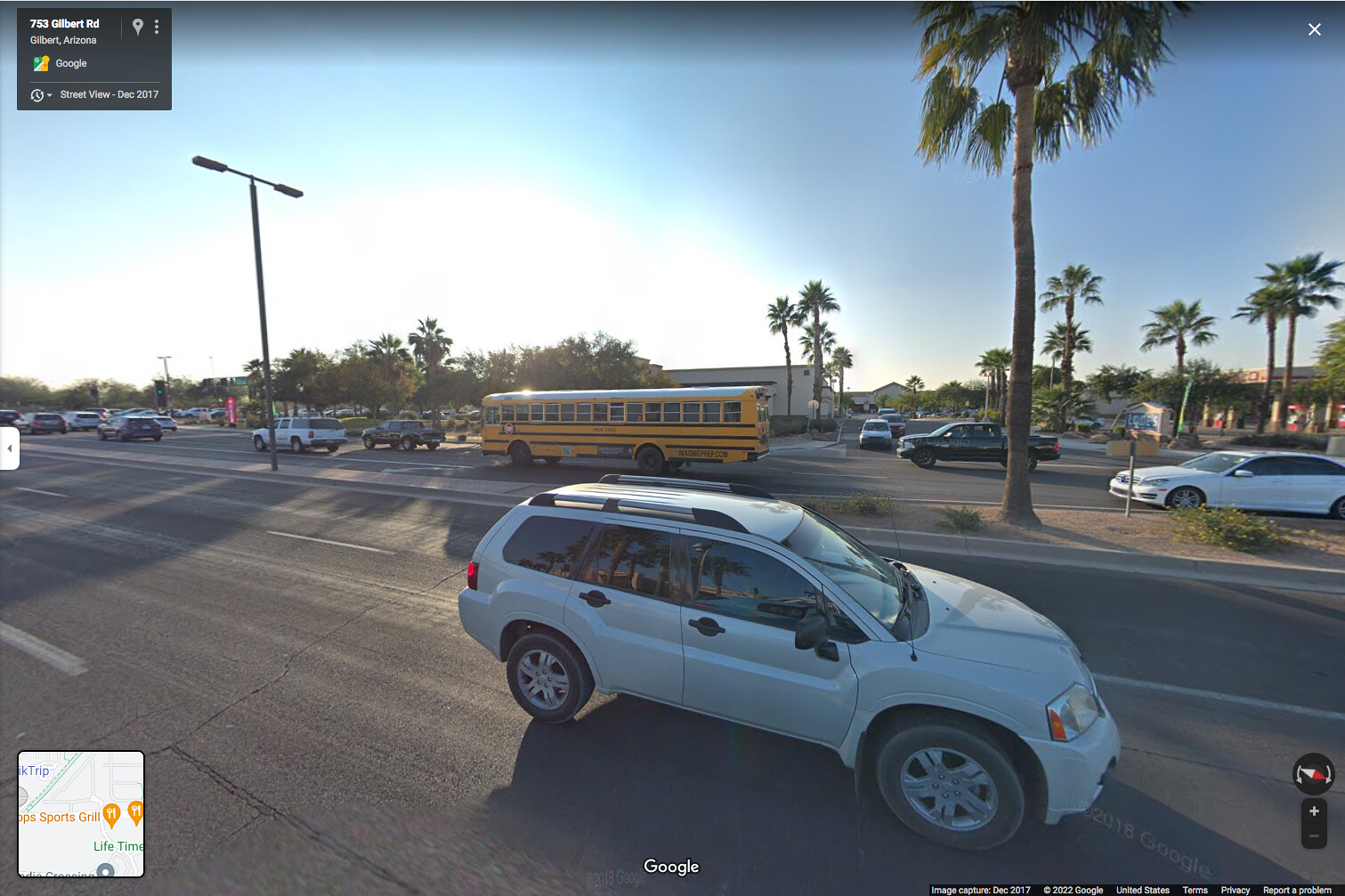The Google Maps Street View image showcases a bustling, multi-lane street scene. The street has at least three lanes in each direction, separated by a central divider. The divider features a large palm tree towards the right side of the frame, accompanied by smaller shrubs. On the left side of the divider, a metallic T-shaped light post is visible, with one light spanning each side of the road.

The bottom center of the image displays the word "Google" in white font. On the left side of the image, a small inset map provides context for the location, revealing the address as 753 Gilbert Road and Gilbert Avenue. This information, along with an icon indicating Google Street View from December 2017, is contained within a black or gray box. The box also features a pin icon and a trio of vertical dots at its top right corner. A white "X" is located at the very top right of the screen, while the bottom right corner displays a compass, a plus and minus button, and a partially obscured black bar with unreadable text.

Several vehicles populate the street. Closest to the viewer, a white van is driving slightly towards us from the side. On the opposite side of the road, an orange school bus, which has a flat front design, leads a line of vehicles: a black truck, a white truck, a black car, and two more cars. Following the school bus is another black truck and a white car. In the background, a parking lot filled with more vehicles is visible, flanked by numerous palm trees that add to the scenic atmosphere. The scene is bathed in the light of a setting sun, with a blue sky and a bright white glow in the middle-right portion of the image, indicating the descending sun.